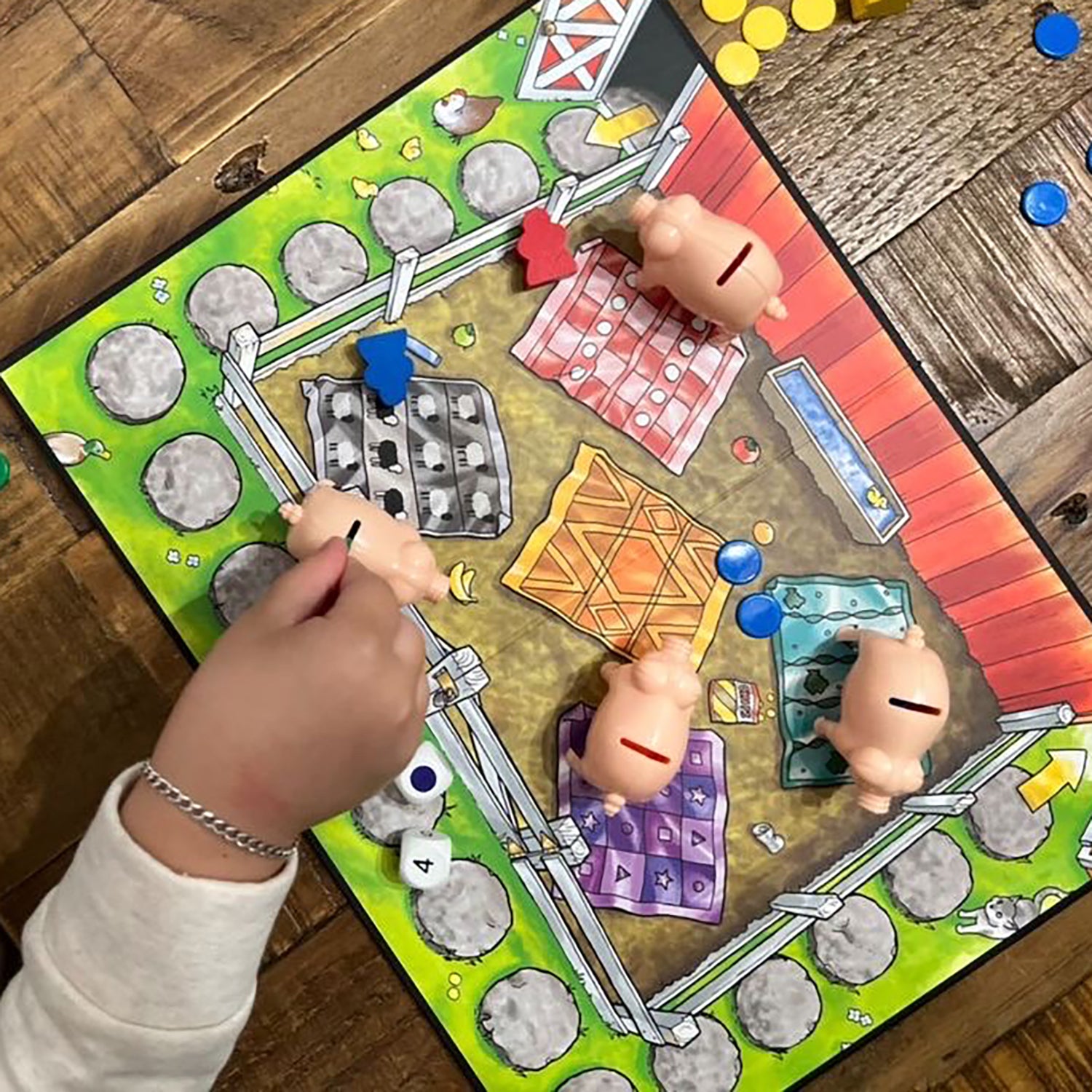In this photograph, a young child is engaging with a detailed board game set on a brown surface, which could either be a table or a floor. The child's right hand, adorned with a bracelet and the cuff of a white shirt, is clearly visible as they interact with the game. The game board depicts a fenced-in barnyard area near a barn, surrounded by a verdant grassy space dotted with white, round stepping stones that trace a path around the pen. The barnyard is encircled by a white fence on three sides.

Inside the barnyard, there are four plastic pigs, each featuring a slot in its back akin to a piggy bank. These pigs rest on colorful squares, possibly representing towels, within the enclosed space. The child's hand is shown placing a coin into one of these piggy banks, emphasizing the interactive nature of the game. There are also colored chips scattered around, notably blue and yellow, likely intended for use with the pigs. Additionally, the game includes dice—one showing the number four and another indicating the color blue.

The vibrant and engaging scene combines elements of a traditional barnyard with the playful concept of piggy banks, creating a whimsical environment for the child to explore. The combination of the green grass, white fence, stepping stones, and various game pieces, along with the visible child's hand, offers a charming snapshot of a moment of play.